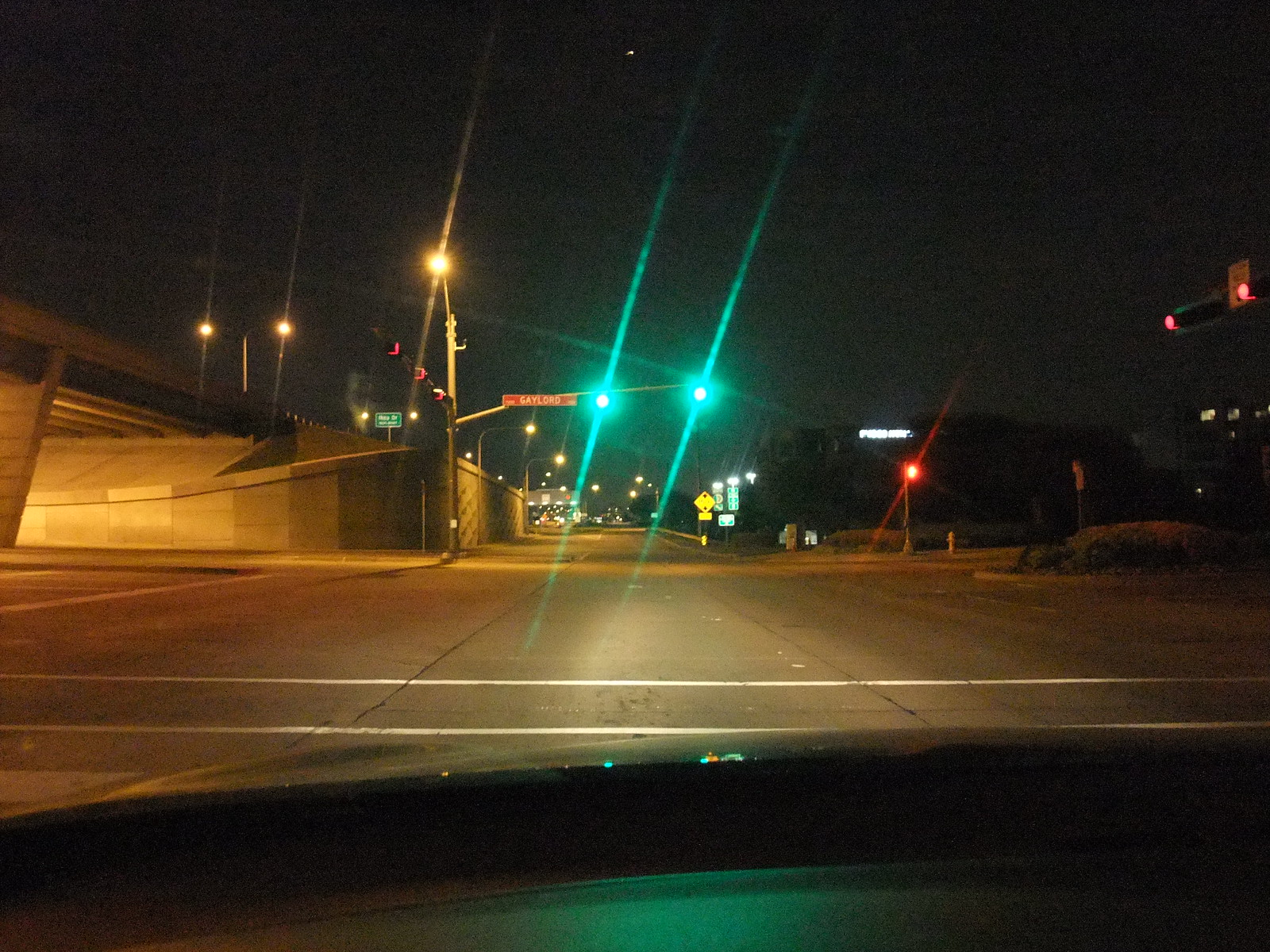A nighttime photograph taken from within a vehicle, possibly through the front or rear windshield. The view is of a deserted intersection, with two green traffic lights aligned horizontally. The vehicle's interior framing is visible around the edges of the image. A red street sign is present but its text is unreadable. Several streetlights illuminate the scene, casting light onto the concrete overpass visible on the left, which features a solid concrete wall underneath. There are no plants or green areas in sight, only a barren sidewalk running beneath the overpass. In the distance, additional streetlights and buildings with illuminated windows can be seen, though none of the details are discernible. The overall atmosphere is quiet and slightly eerie due to the absence of other vehicles or pedestrians.